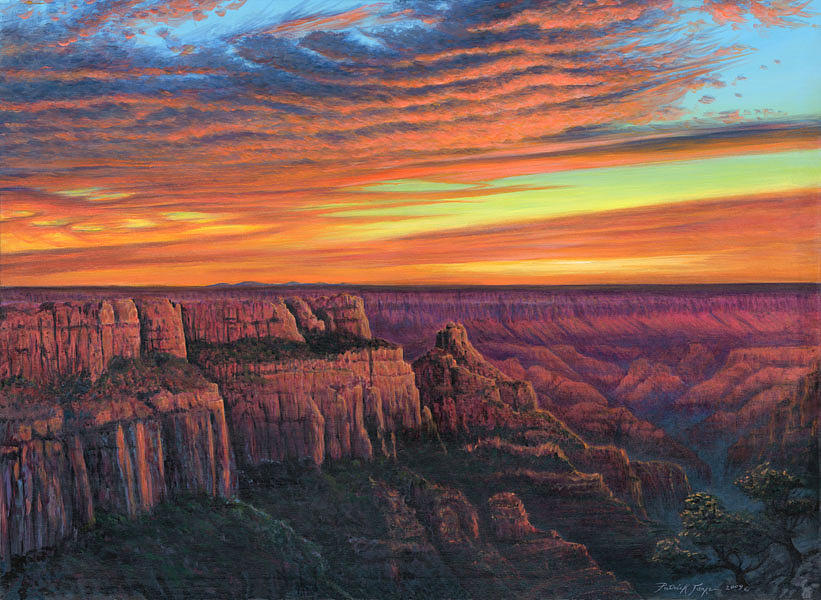This image portrays a stunning landscape that closely resembles the Grand Canyon, featuring a vast expanse of mountains and deep canyons. The cliffs and rocky ledges exhibit a rich palette of brown, reddish, and purplish hues, with shadows enhancing their rugged texture. Lush green grass and sparse vegetation cling to the canyon walls, while big yet distant trees add life to the valley below. A tranquil body of water sits in the bottom right corner, surrounded by greenery. The sky above is a magnificent blend of sunset or sunrise colors, with rippled clouds painting a pattern across a canvas of blue, orange, yellow, and red shades, creating a breathtaking horizon. The painting is signed at the bottom right corner, capturing the essence of this awe-inspiring natural wonder.